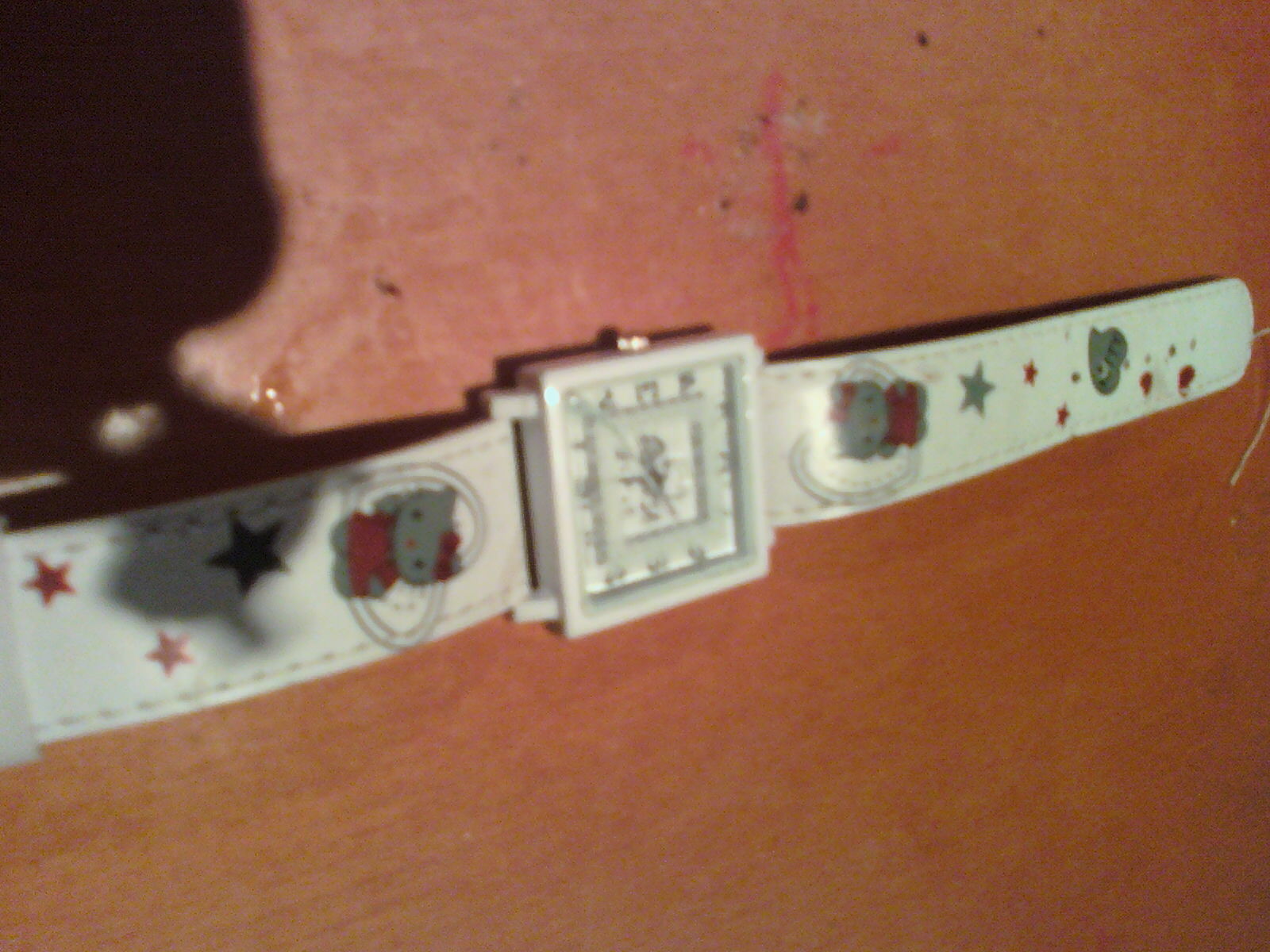An angled view of a white Hello Kitty watch resting horizontally on a dirty, reddish-brown wooden table surface. The watch, which is positioned towards the upper right corner of the photo, features a square face with a smaller inlaid square that houses the hour and minute hands. The blurry watch face and plasticky white band are adorned with Hello Kitty figures at the top and bottom. Stars are scattered along the middle of the band, with another small icon near the bottom. The table surface appears weathered, with a prominent water stain on the left side beneath the watch band and a noticeable red spill in the center of the image, near the top right of the watch band.